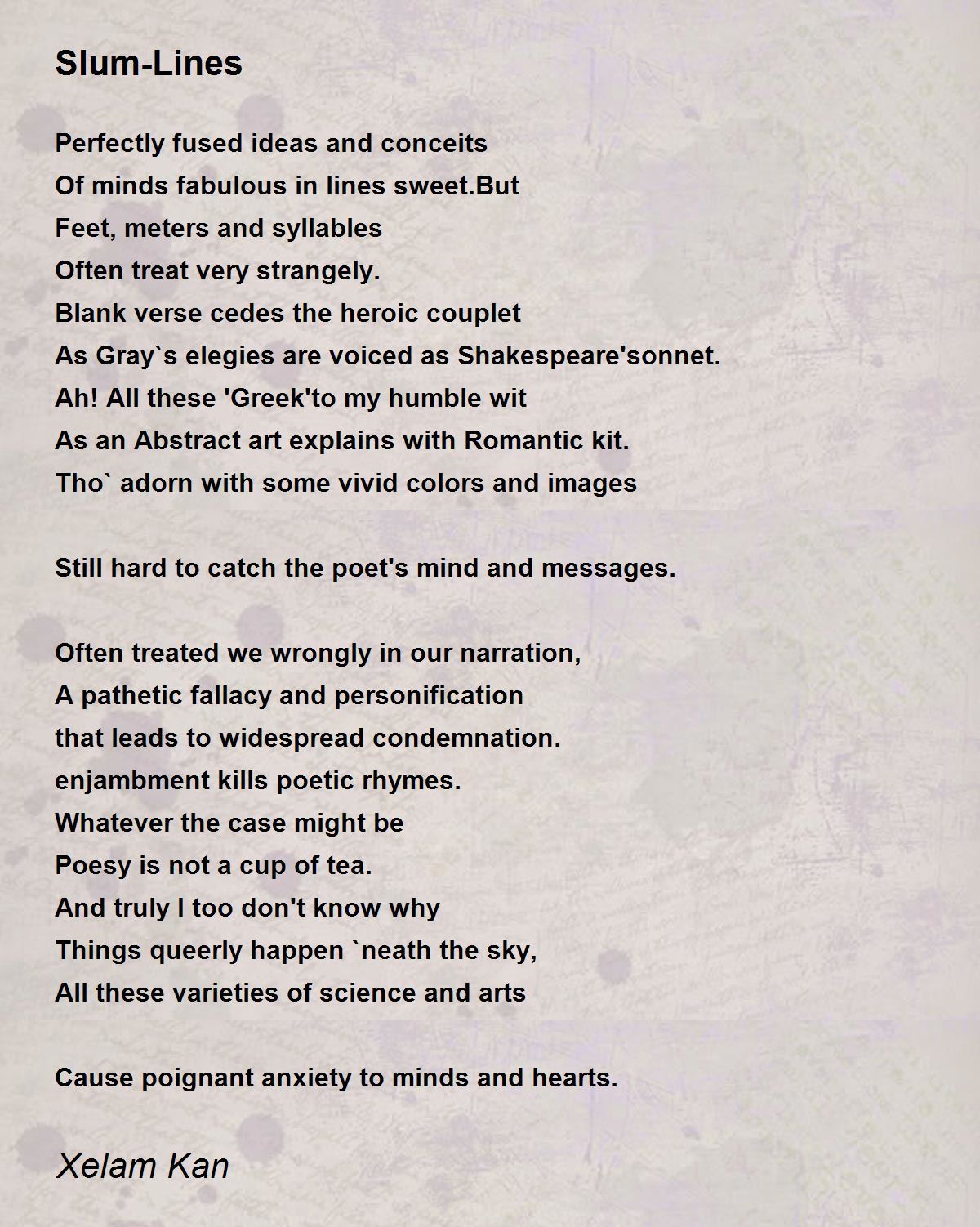This image features a typed poem titled "Slumlines," written by Zeylam Khan. The poem appears on a faded, blotchy, tan-colored paper with subtle, almost translucent cursive text in the background. The poem consists of two full stanzas followed by two standalone lines. The text is presented in a consistent black font with even spacing. 

"Slumlines" explores poetic themes through perfectly fused ideas and conceits. It speaks of minds that are fabulous and lines that are sweet, though often treating feet, meters, and syllables very strangely. Blank verse transitions into heroic couplets, while gray elegies are expressed as Shakespearean sonnets. The poem compares these constructs to abstract art elucidated with a romantic touch, adorned with vivid colors and images. Despite these vivid portrayals, the poet admits to the difficulty in capturing the poet's true intent, often facing misinterpretation and widespread condemnation. Concepts such as pathetic fallacy and personification are touched upon, hinting at the struggles within poetic narration. The concluding lines suggest a resigned contemplation on the elusiveness and complexity of poetry.